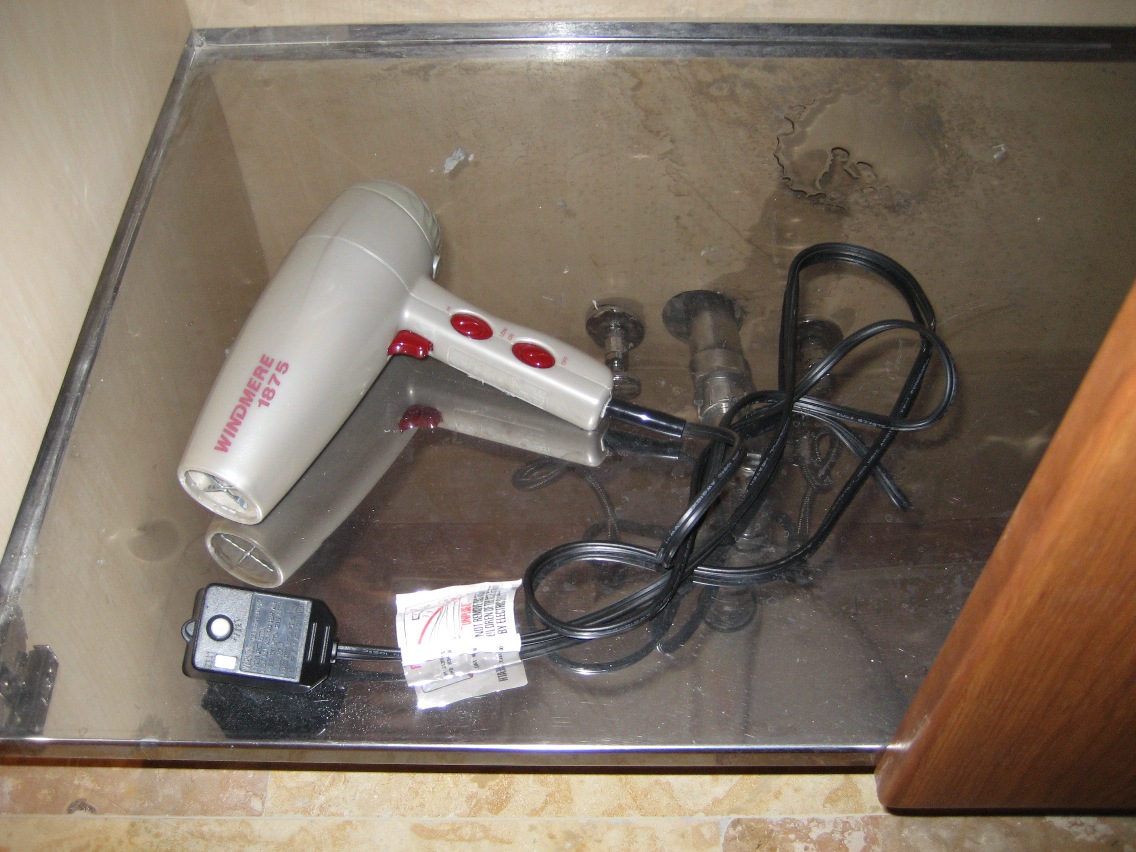This image portrays an old, dirty Windmere 1875 hairdryer, resting on a very dusty and splotchy mirrored base within what appears to be a wooden cabinet. The hairdryer, which has a light gray or silvery hue, prominently features red lettering and three large red buttons—the trigger and two adjustable side buttons. Its tangled black cord has a white safety tag near a rectangular plug with a white button. Surrounding the mirror, there is a brownish, splotchy linoleum floor and a visible wooden panel on the right side, hinting at the structure of the cabinet. The mirror also reflects some piping, adding to the image's aged and unkempt appearance. The scene overall suggests an old, possibly neglected area that may be part of a rundown bathroom or storage space.